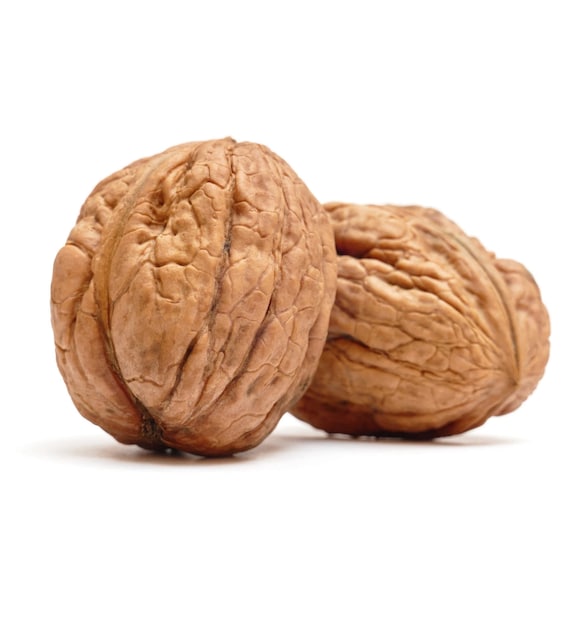This is an extreme close-up photograph of two walnuts, positioned with one slightly in front of the other. The nuts, characterized by their deeply wrinkled and creased light brown shells, are captured in great detail, revealing the intricate craters, dents, and cracks of their outer surfaces. The walnut in the foreground stands more upright, while the one behind leans on its side. Both walnuts cast discernible shadows onto the bright white background, which provides a stark contrast and emphasizes the texture and shape of the nuts.